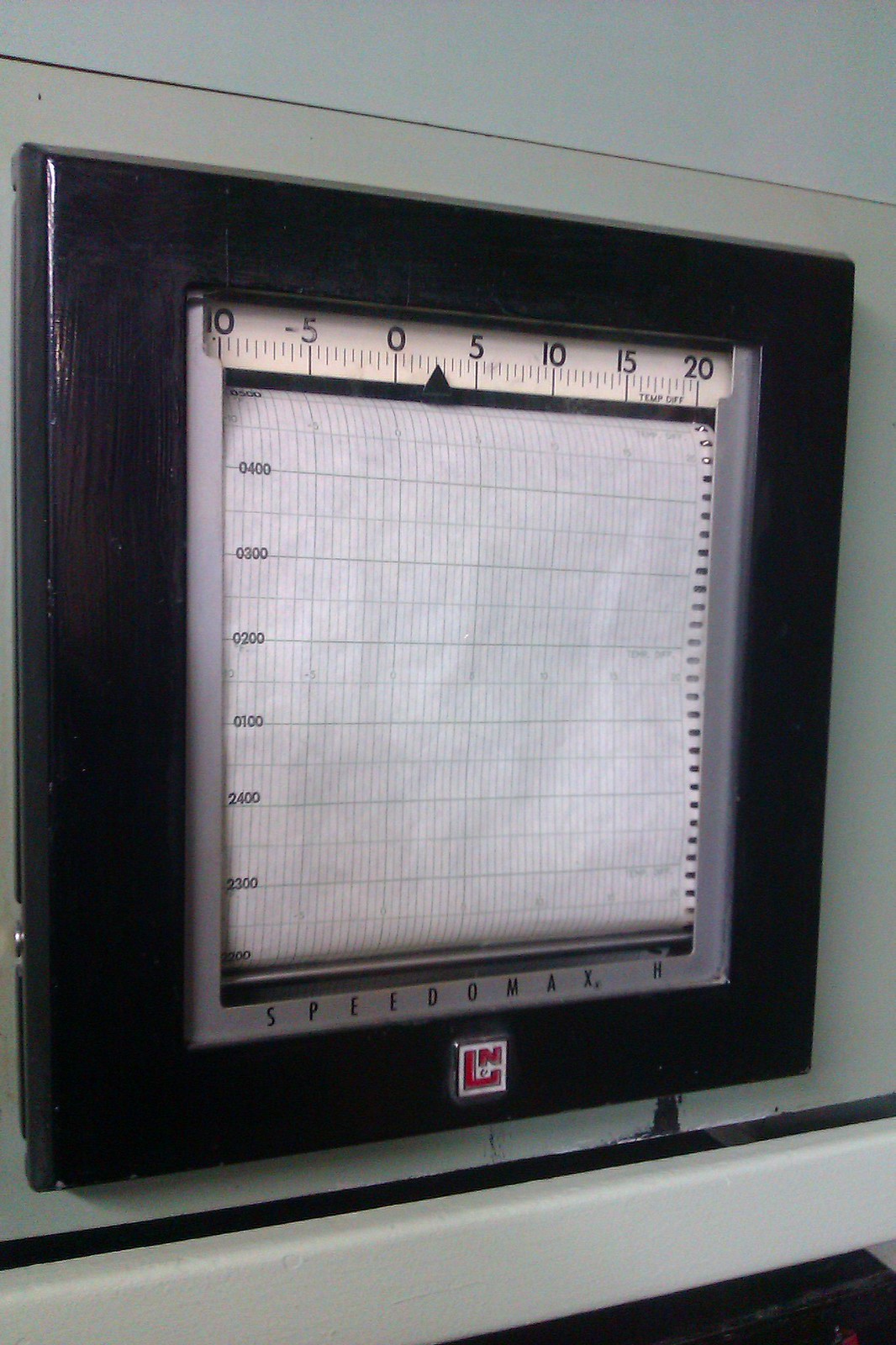The image depicts a black, possibly wooden, framed device that appears to be a timesheet or some form of recording instrument. The frame is square-shaped and has a small white logo at its base. This logo features a red interior outline with another line inside, potentially forming the letters "L" and "N" or "M," all enclosed within a white border.

At the top of the square frame, a ruler-like scale is affixed, marked with increments from -10 to 20, including negative values such as -10 and -5. A black arrowhead is situated between the 0 and 5 marks on this scale.

Below the ruler, a sheet resembling a timesheet is visible. It is printed with times labeled as 04, 03, 02, 01, though the remaining details are difficult to discern. The sheet is overlaid with thin lines. 

At the bottom of the frame, another smaller, silver-colored frame is embedded, displaying the text "Speedomax." 

The entire assembly is mounted against a white wall or another white surface. The design and intricacies suggest a sophisticated measuring or recording instrument.